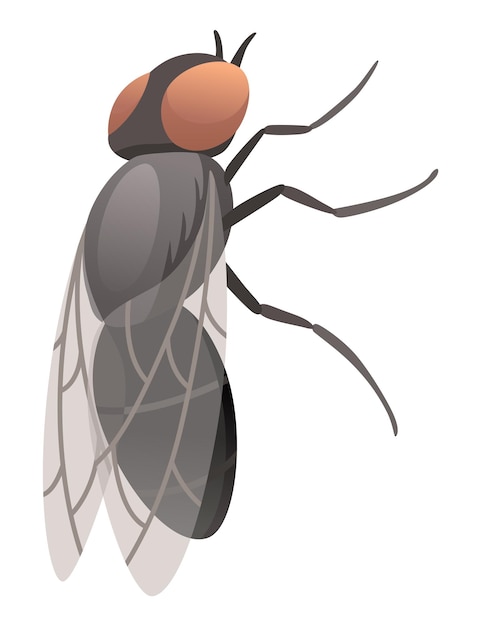This image is a detailed, vertically aligned, computer-generated illustration of a fly, set against a white background. The portrayal offers a zoomed-in perspective, presenting a top and slightly right-side view. The insect features strikingly large, burnt orange eyes dominating the upper part of the head, with a distinct black stripe running down the middle. Two prominent black antennae extend from the top of the head. The body of the fly is a dark, charcoal gray, accented with lighter gray markings along the top. Its wings are long, stretching from the head past the end of its body, and are translucent with intricate, branching darker gray veins. The insect's black legs are visible, splaying outwards to cling to an invisible wall, transitioning to gray at the tips. Three legs are noticeable on the right side, offering a detailed view of the fly's anatomy.